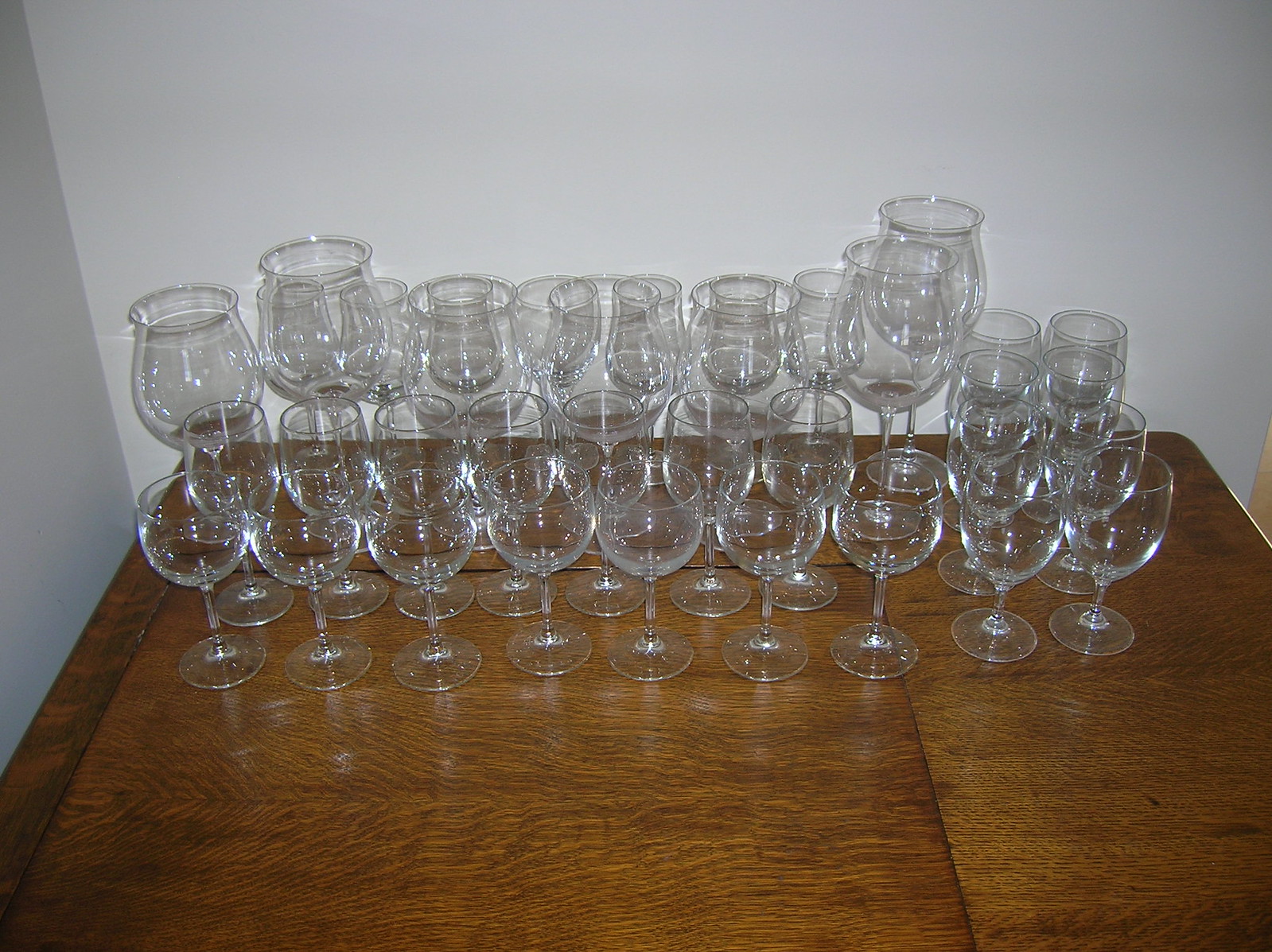This is a detailed photograph of a neatly arranged assembly of champagne and wine glasses placed on a beautiful, striped oak or tiger oak rectangular wooden table. The setting is pushed into the corner of a room with simple, white-painted walls. The glasses are organized in rows: the front row contains nine glasses, followed by another row of nine. Further back, there is a row of taller glasses, amounting to a similar number, and at the very rear, a row of slightly shorter glasses, contributing to a total count of around 40 to 50 glasses. Each glass is made of clear, transparent glass, and their arrangement is meticulously even and symmetrical, creating a visually appealing, almost geometric display on the wooden surface.